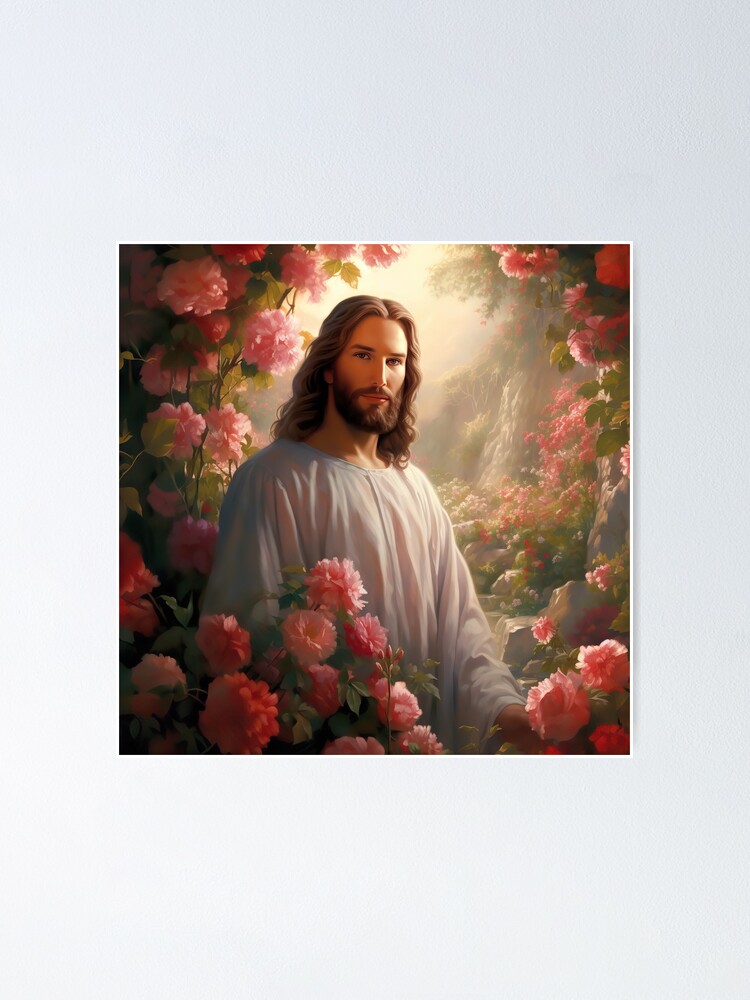In the center of this square-shaped image is a painting or digital creation of Jesus. Depicted with long, wavy brown hair, a bird-like moustache, and a brown beard, Jesus has pale skin and is adorned in a loose-fitting, sheer white robe. Only his face and upper body are visible. Surrounding Jesus is a circle of pink carnations set against a backdrop of green leaves, suggesting an outdoor scene that is bright and well-lit. The entire composition is framed by a thick, pale blue border, which is notably thicker at the top and bottom and thinner on the sides. Jesus is positioned looking forward, as if towards a camera, at the center of this detailed, nature-immersed portrayal.